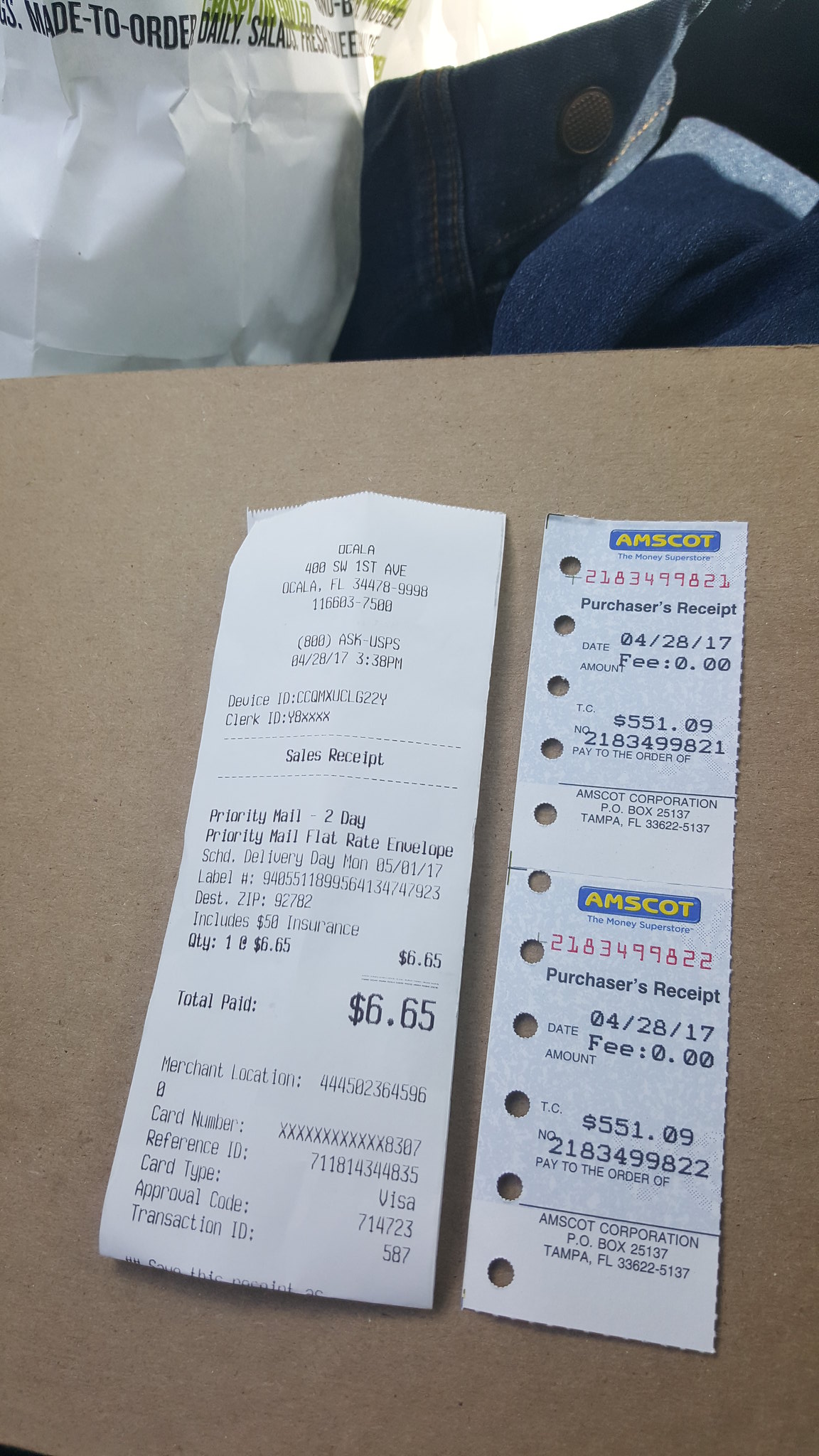In this photograph, two white receipts are laid out side by side on a table. The receipt on the left shows a total amount paid of $6.65, which was settled using a Visa credit card. The approval date on this receipt is July 14, 2023, with a transaction ID of 587. Some details on this receipt are difficult to make out, but an address is visible at the top. The right-hand receipt is slightly narrower and features uniform punch holes running down its left side. The name of the store, "AMSCOT," is prominently displayed at the top, followed by the word "receipt."